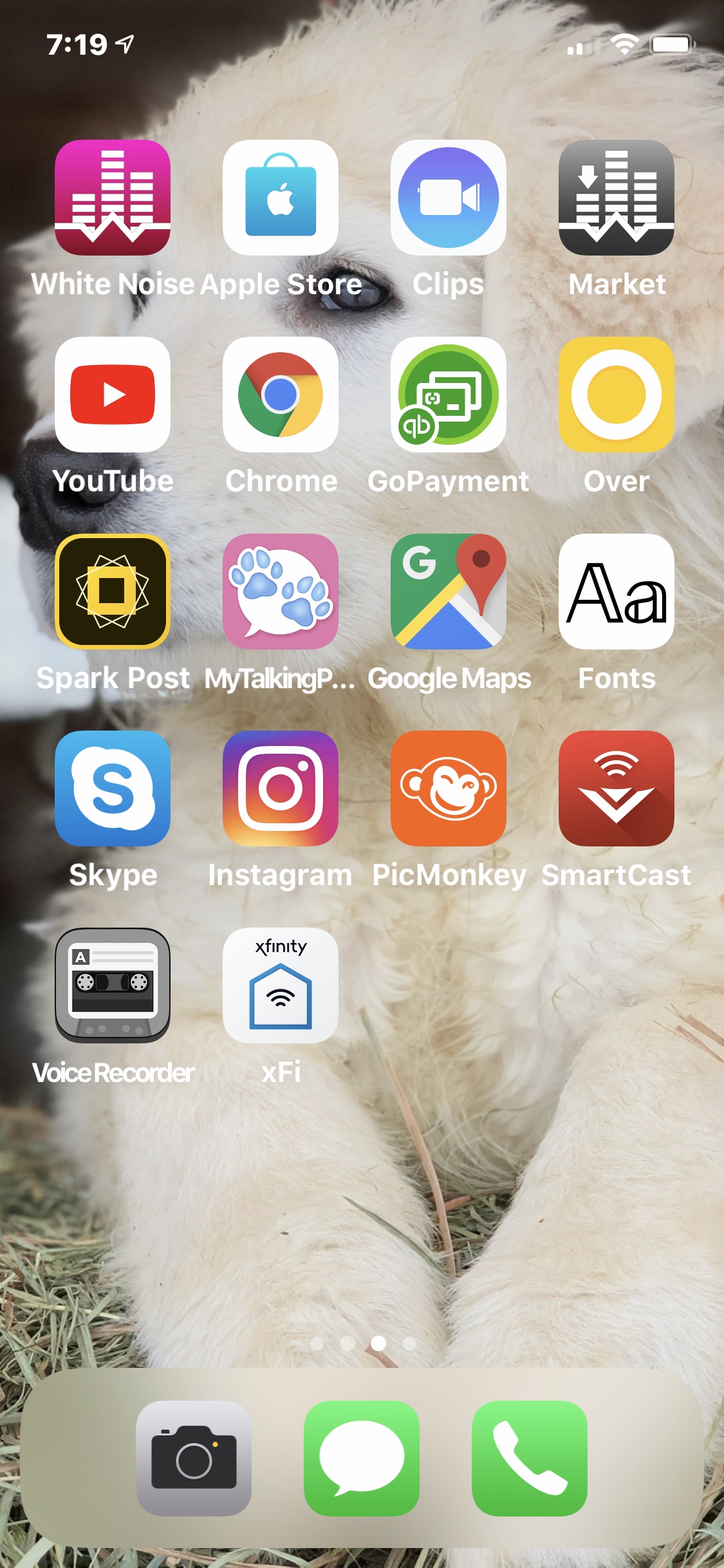The image showcases the front interface of a cell phone against a black background. Prominently featured is an adorable, fluffy white puppy nestled comfortably on a bed of hay, exuding cuteness. The puppy's black eye peeks out from the surroundings, but its full face isn't visible. The screen displays various app icons including White Noise, Apple Store, Clips, Market, YouTube, Chrome, GoPayment, Over, SparkPost, MyTalkingSomething, Google Maps, Fonts, Skype, Instagram, PickMoney, SmartCast, Voice Recorder, and X-Fi. At the bottom of the screen, a silver circle contains icons for the camera, messages, and telephone, with the latter two represented in green circles.